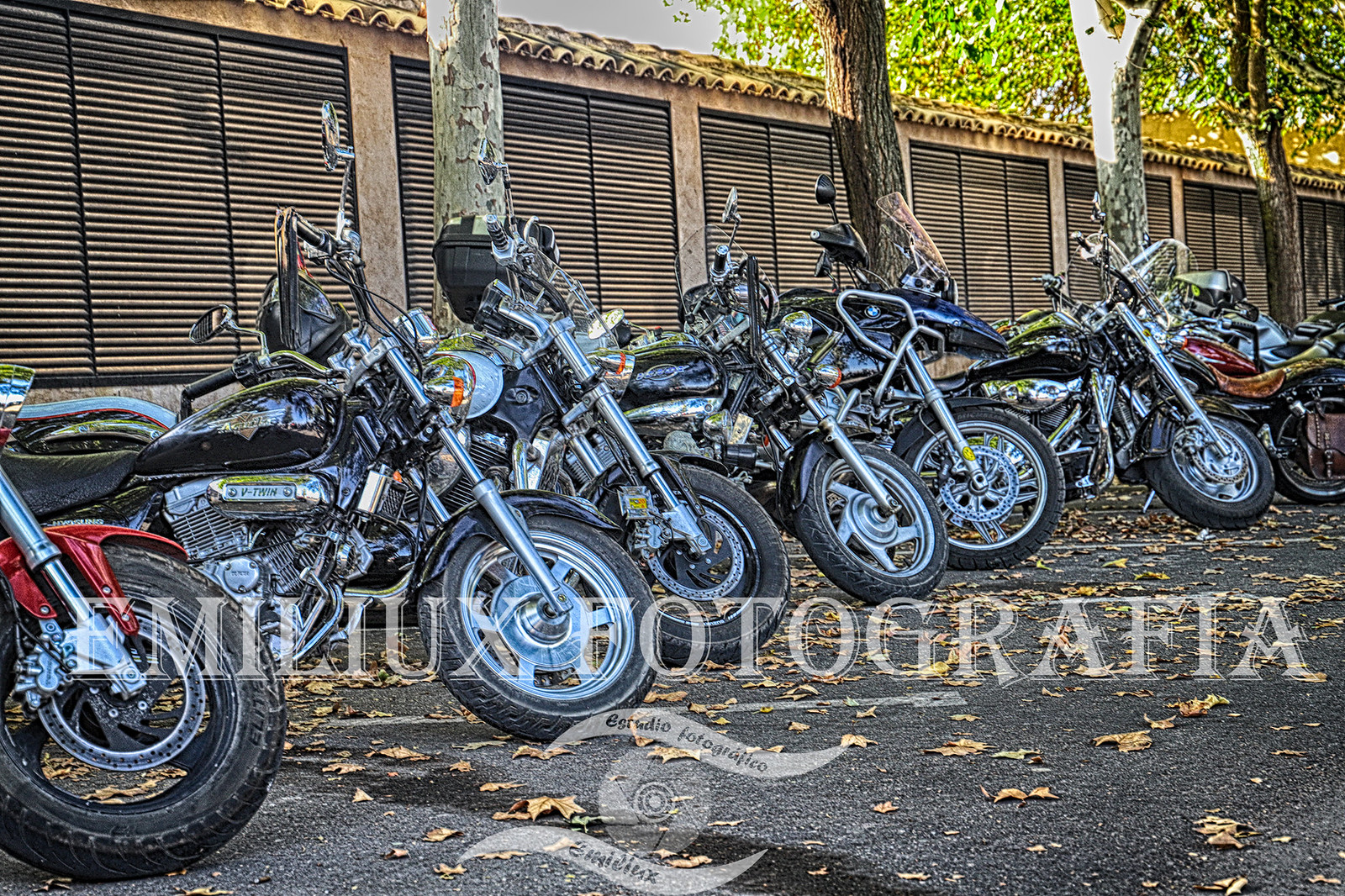This horizontal, realistic photograph captures a lineup of several motorcycles parked on asphalt in what seems to be a well-lit outdoor setting. The vibrant green leaves of the trees in the background suggest good sunlight despite the light gray sky above. A beige building with light tan tile roofs and what appear to be black screens or possibly roll-up garage doors stands behind the trees. 

In the foreground, we see between six to eight motorcycles, all with their front wheels pointing towards the right. The bikes are in various colors including black, blue, silver, red, and potentially yellow. Notably, one of the motorcycles displays a BMW emblem, highlighting the diversity of models present. Dead leaves are scattered across the asphalt, adding to the scene's natural ambiance.

Positioned centrally in the photograph is a watermark in transparent white text that reads "Emilio X Fotografia," adding a professional touch to the image. The picture was likely taken from a leftward angle, providing a slight 45-degree view of the motorcycles, which are visibly leaning to the side. The motorcycles benefit from the orderly arrangement, creating a visually appealing and detailed composition.